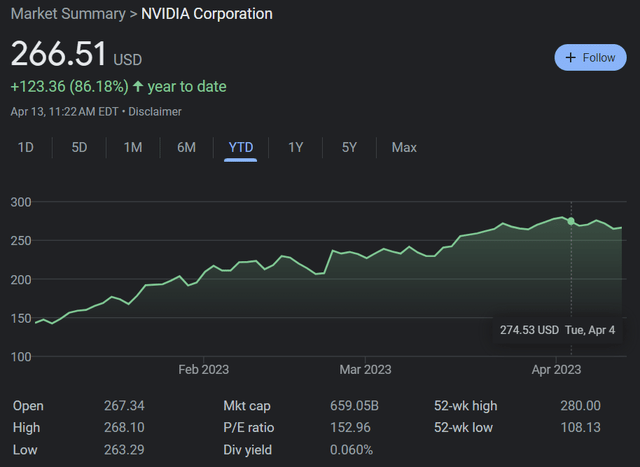**Screenshot Description:**

The image is a screenshot featuring a black background. In the upper left-hand corner, the text "Market Summary" appears in gray, followed by a greater-than sign. Immediately after, "NVIDIA Corporation" is prominently displayed in white.

Directly below, the large white number "266.51" indicates a value, and to its right, the text "USD" appears in smaller gray all-caps. 

On the right side of this section, there is a blue oval "Follow" button. 

The next line down shows a green plus sign followed by "123.36" and "86.18%" inside parentheses, indicating a positive change. A green upward arrow accompanies the text "Year to Date."

Below this, in smaller gray text, the date "APR 13, 11:22 A.M. EDT" is noted, followed by the word "Disclaimer."

Further down, there are black boxes featuring various time frames in gray text: "1D, 5D," followed by "1M, 6M," with "YTD" highlighted in blue and underlined, and then "1Y, 5Y, Max."

Beneath these options is a graph. The left side has numbers in gray: "300, 250, 200, 150, 100," with horizontal light gray lines running across the graph. The graph line itself is green.

At the bottom, headings like "February 2023, March 2023, April 2023" are aligned horizontally. Below these, on the left side, words in white text say "Open," "High," "Low," followed by columns of corresponding numbers on the right. Additional columns of numbers are located at the bottom of the screenshot.